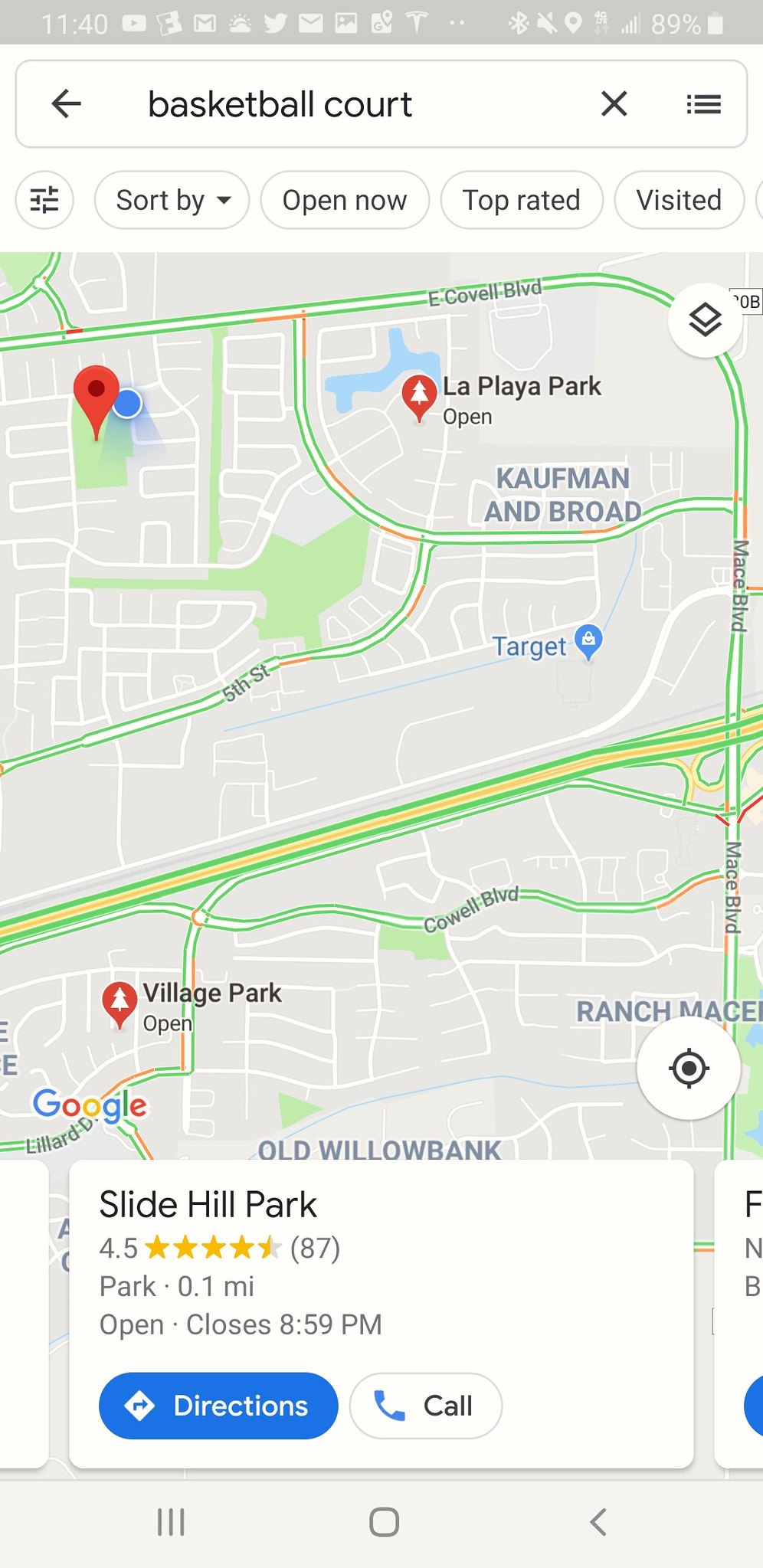A smartphone screenshot displays Google Maps directions for a search query for a basketball court. The search bar at the top contains the typed query "basketball court". Below the search bar, the screen shows a map with the specified route to the basketball court. The map prominently features a red Google Maps pin marking the location of Slide Hill Park, which is the nearest court, standing just 0.1 miles away. A blue circle indicates the user's current location. The park is noted for its high rating of 4.5 stars and is open until 8:59 PM. The map also displays surrounding roads, including East Covell Boulevard and Mace Boulevard, highlighted in green for better navigation.